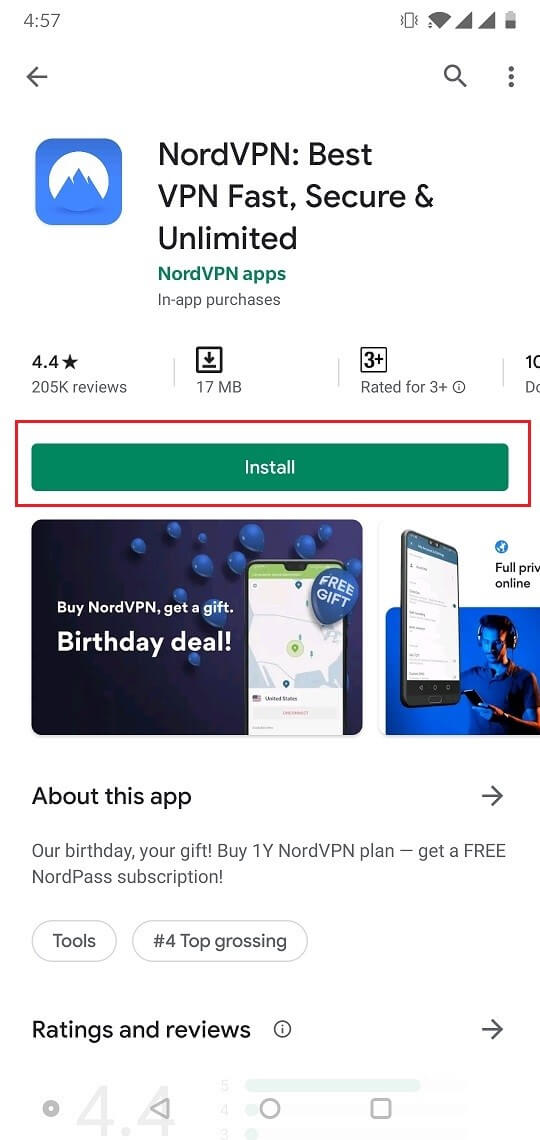Here's a detailed and cleaned-up caption for the image:

---

The screenshot displays a cell phone screen. In the upper left corner, the time is shown as "5:57". On the upper right, the phone is set to Vibrate mode, and icons indicate active Wi-Fi, data, and cell signal. The battery level is around 50%. Just below, there is a left arrow, a search icon, and a vertical ellipsis (three dots) on the right.

Immediately below this is the text "NordVPN. Best VPN, fast, secure, and unlimited," accompanied by a blue square logo featuring a white circle with blue mountains inside it to the left. To the right, green text reads "NordVPN apps," followed by "in-app purchases" in smaller lettering underneath.

Below this section, the app's rating is displayed as 4.4 stars based on 205,000 reviews, with a note that the download size is 17 megabytes. The app is rated for users aged 3 and up, but part of this rating is cut off by the image border. 

Further down, there is a long, thin green button with white "Install" text, highlighted by a red box added through photo editing. 

Beneath this, promotional text reads: "Buy NordVPN, get a gift, free, get a gift, birthday deal." On the right, partially visible text says "full PRIV online", which is also cut off. 

Finally, there is an "About this app" section mentioning: "Our birthday, your gift. Buy one year NordVPN plan, get a free NordVPN pass subscription."

---

In this updated caption, the detailed description of each section of the screenshot has been preserved and formatted to make it clear and easy to understand.